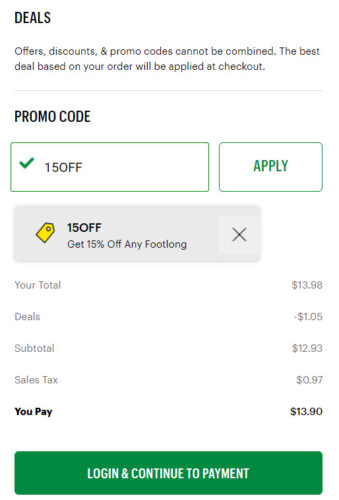This screenshot captures a mobile checkout screen. Prominently, in the top left corner, there's a header labeled "Deals." Just below, in grey text, there's a note explaining that offers, discounts, and promo codes cannot be combined and that the best deal based on the order will be applied at checkout. Underneath, the section titled "Promo Code" features a green checkbox marked with "15 off" alongside a green checkmark. To the right, a button outlined in green with the word "Apply" in green text is visible. Below this, a tag indicating "15 off" offers 15% off any footlong sandwich.

The order's price breakdown follows: 
- Total: $13.98
- Deals: -$1.05
- Subtotal: $12.93
- Sales Tax: $0.97
- Final Amount: $13.90

All totals are in grey, except "You Pay $13.90," which stands out in black. At the bottom of the screen, a large green button with white text reads, "Login and Continue to Payment." The screen appears to show a food order, specifically a footlong sandwich, with a discount applied using a promo code.